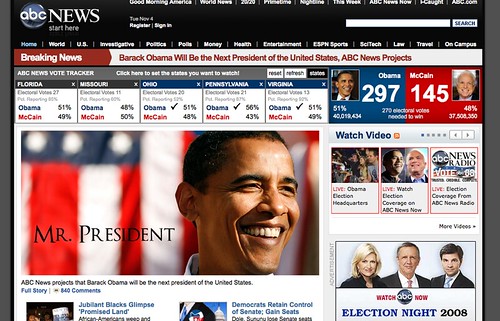This image is a detailed screenshot of the ABC News Network homepage, highlighting significant elements surrounding the 2008 Presidential Election. Dominating the interface is a black banner across the top with white text links that, despite their small size, are organized under different sections, including "Good Morning America," "World News," "Investigative," "Politics," "Polls," "Money," "Health," "Entertainment," "ESPN," "Sports," "Sci-Tech," "Law," "Travel," and "On Campus." A search bar is also integrated into this black band for user convenience.

A striking red banner stretches horizontally across the center of the screenshot, boldly announcing in white text: "Breaking News - Barack Obama will be the next President of the United States, ABC News Projects." Below this proclamation, the election results are prominently displayed, showing Obama securing 297 electoral votes against McCain's 145. Additional statistics break down results from key states such as Florida, Missouri, Ohio, Pennsylvania, and Virginia.

On the left side of the page, a large, captivating image features Barack Obama celebrating with a jubilant expression. The caption "Mr. President" accompanies the image, while the background proudly showcases the American flag, underscoring the momentous occasion. Adjacent to this, an unobtrusive ad on the lower right-hand side of the screen reminds viewers that this moment is from "Election Night 2008."